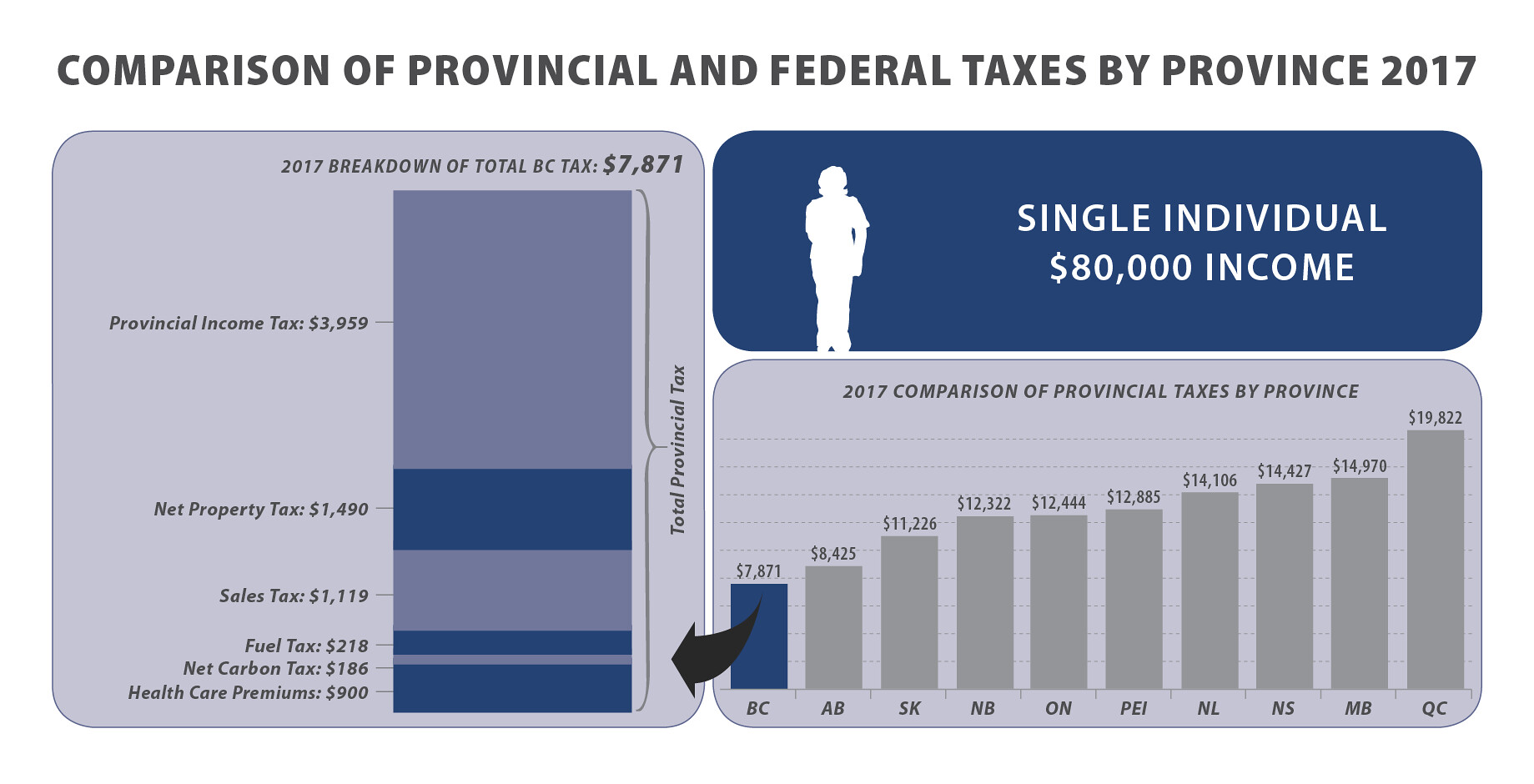The image titled "Comparison of Provincial and Federal Taxes by Province, 2017" presents a detailed breakdown of taxes for a single individual with an $80,000 income from the province of British Columbia (BC). On the left side, a rounded rectangle labeled "2017 Breakdown of Total BC Tax" details taxes amounting to $7,871, comprising Provincial Income Tax ($3,959), Net Property Tax ($1,490), Sales Tax ($1,119), Fuel Tax ($218), Net Carbon Tax ($186), and Health Care Premiums ($900). This compartmentalized column graphically illustrates the contribution of each tax category. To the right, another rounded rectangle features a silhouette of a person, and the accompanying bar graph compares provincial taxes across ten provinces, from BC (the lowest at $7,871) to Quebec (QC, the highest at $19,822) without detailing individual tax components for other provinces. The bar graph emphasizes BC's comparatively lower tax burden.